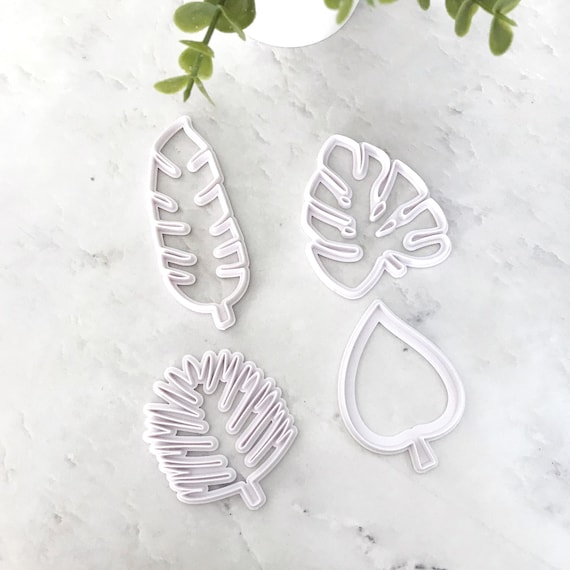This detailed image features four distinct white plastic leaf-shaped cookie cutters arranged on a textured white marble background. At the top of the image, partially visible, is a round, white planter with small, round green leaves extending into the frame. The leaf cutters, all facing to the left, are prominently showcased in the center. 

- The top left cookie cutter is an elongated, oval shape with five ridges on each side to depict the veins.
- The top right cutter has a stubby, heart-shaped silhouette, featuring three deep ridges on both sides to form its veins.
- Positioned below this, the bottom right cutter is a simple heart shape without any vein detailing.
- To the left of this, the bottom left cutter has a rounded, almost circular form with numerous deep ridges, possibly eight or nine, representing its vein structure.

Each cutter represents different leaf types, and while they could be used for cookies, they might also serve as molds for other crafts like resin or wax. The blending of fine details emphasizes the variety and utility of these cutters against the nuanced marble backdrop.